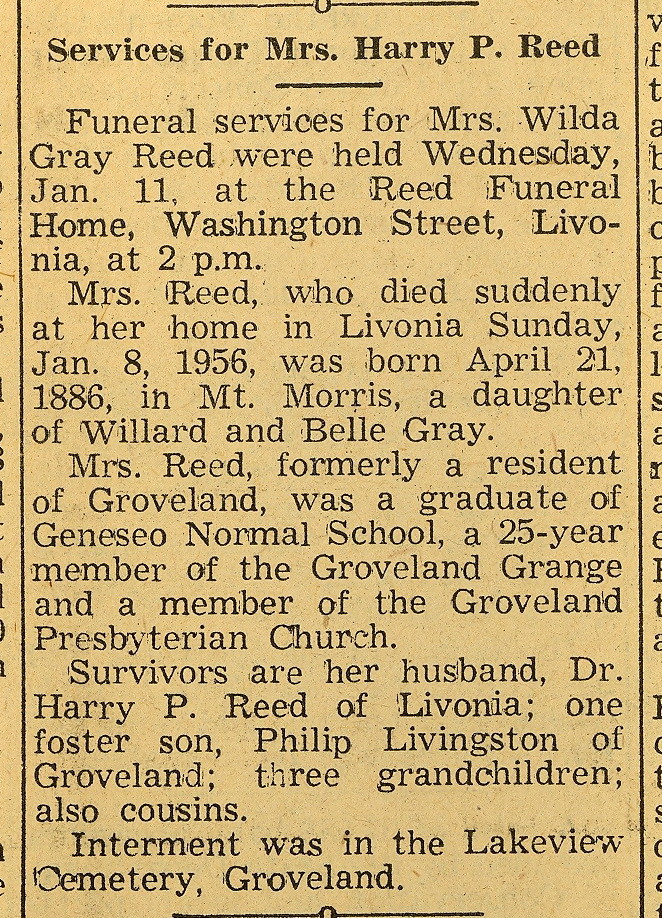The image is an aged snippet from a sepia-toned newspaper, showcasing an obituary titled "Services for Mrs. Harry P. Reed" in prominent black font. It documents the funeral services for Mrs. Wilda Gray Reed, which took place on Wednesday, January 11, 1956, at the Reed Funeral Home on Washington Street in Livonia, at 2 p.m. Mrs. Reed, who passed away suddenly at her home on Sunday, January 8, 1956, was born on April 21, 1886, in Mount Morris. She was the daughter of Willard and Belle Gray. A former resident of Groveland, Mrs. Reed graduated from Geneseo Normal School, was a 25-year member of the Groveland Grange, and belonged to the Groveland Presbyterian Church. She is survived by her husband, Dr. Harry P. Reed of Livonia, a foster son, Philip Livingston of Groveland, three grandchildren, and several cousins. Her interment was held at Lakeview Cemetery in Groveland.